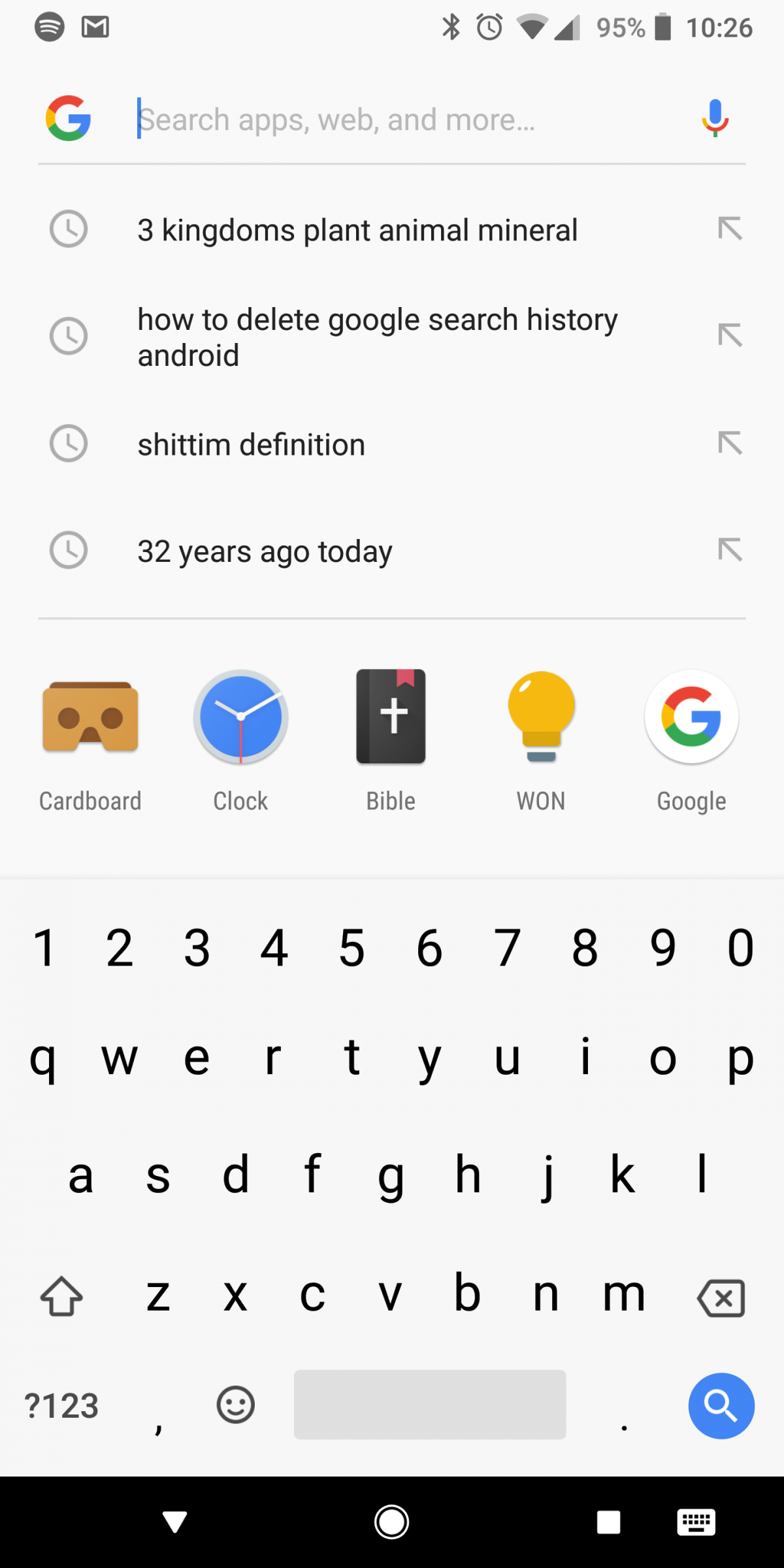The image shows a smartphone screen with various icons and text. In the upper left corner, there are three horizontal lines and a circle icon, possibly a menu and notification indicator. An envelope icon is also visible, likely denoting email notifications. On the upper right, the status bar displays a Bluetooth icon, an alarm clock, Wi-Fi signal bars, cellular signal bars, a battery indicator at 95%, and the time reading 10:26.

Below the status bar, on the left side, there's the colorful "G" logo of Google in red, yellow, green, and blue. Next to it, the text "Search Apps, Web, and More" appears in gray. On the right side of this bar, there's a microphone icon in Google’s colors.

Below this, a gray line separates the next section, which lists four recent search items. Each item has a small gray clock face icon to the left of black font text. The items are titled "Three Kingdoms, Plant, Animal, Mineral," "How to Delete Google Search History Android," "Shittim Definition," and "32 Years Ago Today." Each title is accompanied by an upward-pointing arrow on the right.

Further down, another gray line separates this section from the next, which reads "Cardboard," "Clock," "Bible," "Wand," "W-O-L-N," and "Google." Each of these entries has its respective icon beside it.

At the bottom of the screen, a virtual keyboard with a white background and black letters and numbers is visible. The keys are not individually marked out, and there is a blue search button included.